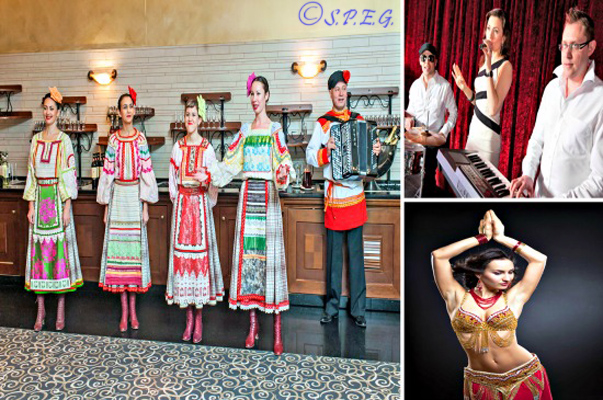This collage features three distinct photographs. The largest image on the left showcases four women dressed in colorful, traditional European attire with slicked-down hair, each adorned with a flower matching their vibrant aprons. They stand in a line in front of a wooden cabinet filled with various bottles, possibly indicating a bar setting. The women's outfits include white as a base color with multi-colored aprons: one green with bright pink flowers, another white with a red center, and another featuring a pattern of bold black, green, and red stripes. They all wear red boots. Beside them stands a man dressed in black pants, a tunic-like colored shirt, and a distinctive hat adorned with a red ball or flower, playing an accordion.

In the top right photo, a Caucasian man with glasses and a close-cut hairstyle is playing a keyboard. He wears a white shirt. Beside him, a woman in a white dress with black stripes sings into a microphone, while another man in the background, wearing sunglasses and a hat, possibly a black beret, watches.

The bottom right image features a belly dancer with dark hair, posed with her hands forming a triangle above her head and her hip thrust to the right. Her attire includes a bikini top, showcasing her midriff, and a long, flowing skirt, both embellished with gold and red.